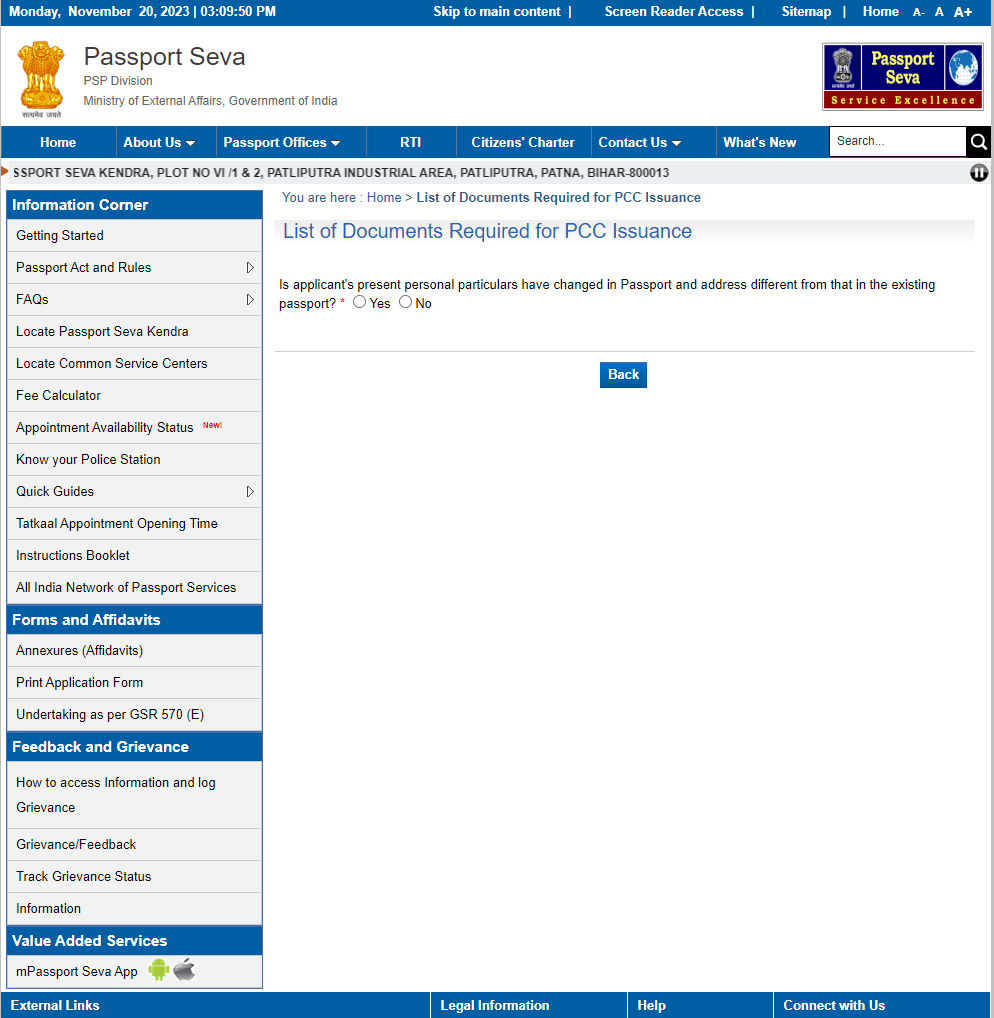Screenshot of Passport Sewa Website taken on Monday, November 20th, 2023 at 3:09:50 PM

This image captures the detailed interface of the Passport Sewa (PSP Division) website under the Ministry of External Affairs, Government of India. The top navigation bar includes links for 'Skip to main content,' 'Screen Reader Access,' 'Sitemap,' 'Home,' and options to modify font size. The header prominently displays that this is part of the Passport Sewa Service Excellence initiative, likely providing passport-related services.

The primary horizontal menu, from left to right, features tabs such as 'Home,' 'About Us,' 'Passport Offices,' 'RTI,' 'Citizens Charter,' 'Contact Us,' 'What's New,' and a 'Search' bar.

On the left side, a vertical menu is categorized into several sections:

1. **Information Center:** 
   - Getting Started
   - Passport Act and Rules
   - Frequently Asked Questions
   - Locate Passport Sewa Kendra
   - Locate Common Service Centers
   - Fee Calculator
   - Appointment Availability Status (marked as new)
   - Know Your Police Station
   - Quick Guides
   - Tatkal Appointment Opening Time
   - Instruction Booklet
   - All India Network of Passport Services

2. **Forms and Affidavits:**
   - Affidavits
   - Print Application Form
   - Undertaking as per GSR 570E

3. **Feedback and Grievance:**
   - How to Access Information and Log Grievance
   - Grievance/Feedback
   - Track Grievance Status
   - Value-Added Services

4. **M Passport Sewa App:**
   - Available on Android and Apple platforms.

At the bottom of the page, links for 'External Links,' 'Legal Information,' 'Help,' and 'Connect with Us' are visible.

The currently displayed content indicates that the user is in the section titled "You are here: Home > List of Documents required for PCC issuance," which also lists conditions regarding changes in personal particulars and different addresses from the existing passport, with options to answer 'Yes' or 'No' and to go back.

Overall, this screenshot illustrates a comprehensive user interface aimed at facilitating various passport-related services for customers, and possibly employees, of the Indian government.